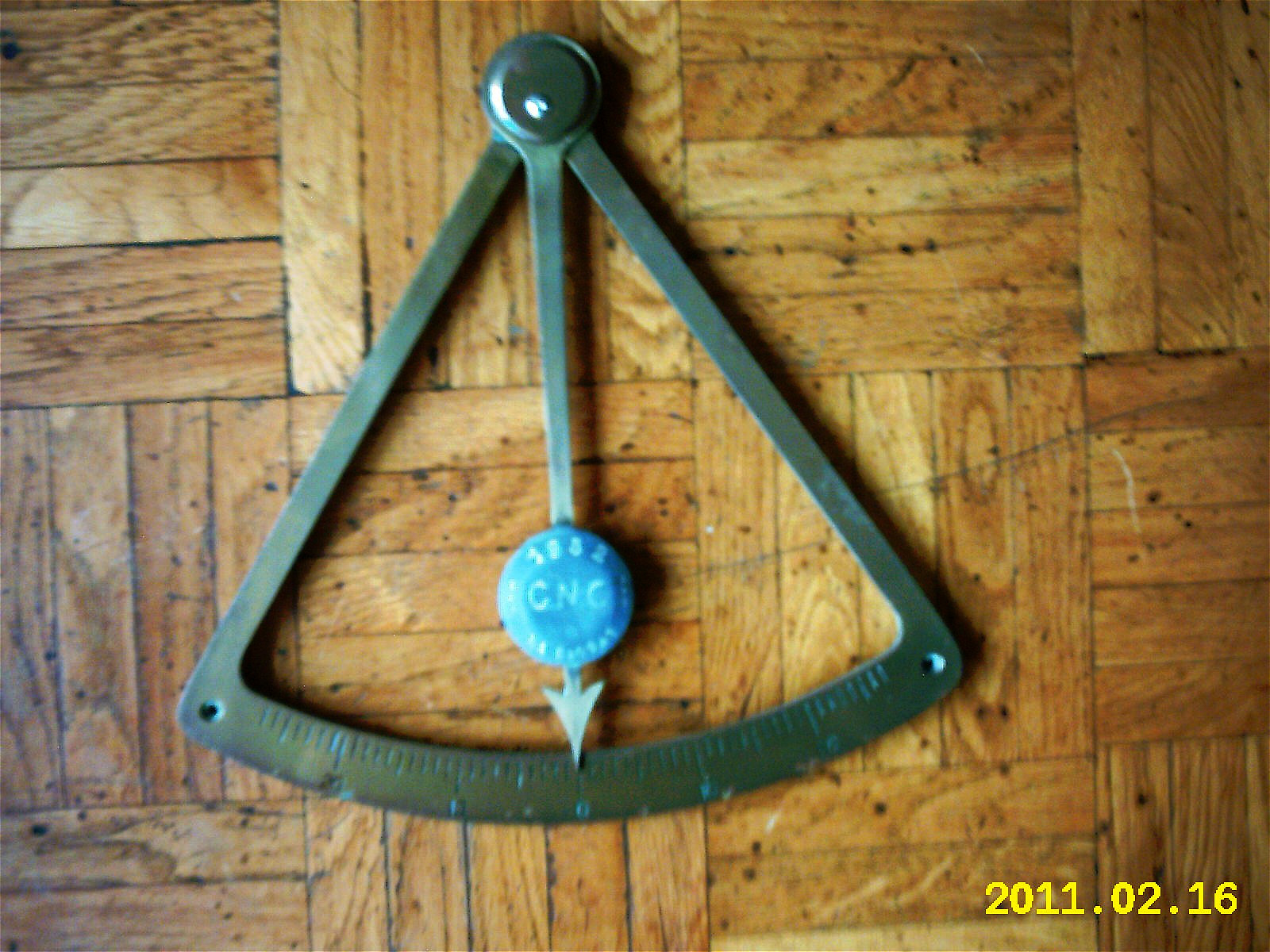The image depicts an old maritime navigation tool, commonly known as a protractor, fashioned from metal. It is triangular in shape with a curved base that features etched markings resembling a ruler, enabling precise measurements. An arrow or pointer is affixed to a dial at the top and moves across the plane, currently positioned at the zero mark in the center of the scale. This pointer is enhanced with a circular blue marking or cap, inscribed with "CNC 1982". The protractor rests against a crafted wooden surface, where wood blocks are arranged alternately in a horizontal and vertical pattern. In the bottom right corner, a date is printed in yellow text, reading "2011.02.16", likely added by a digital camera at the time of capturing the photograph.